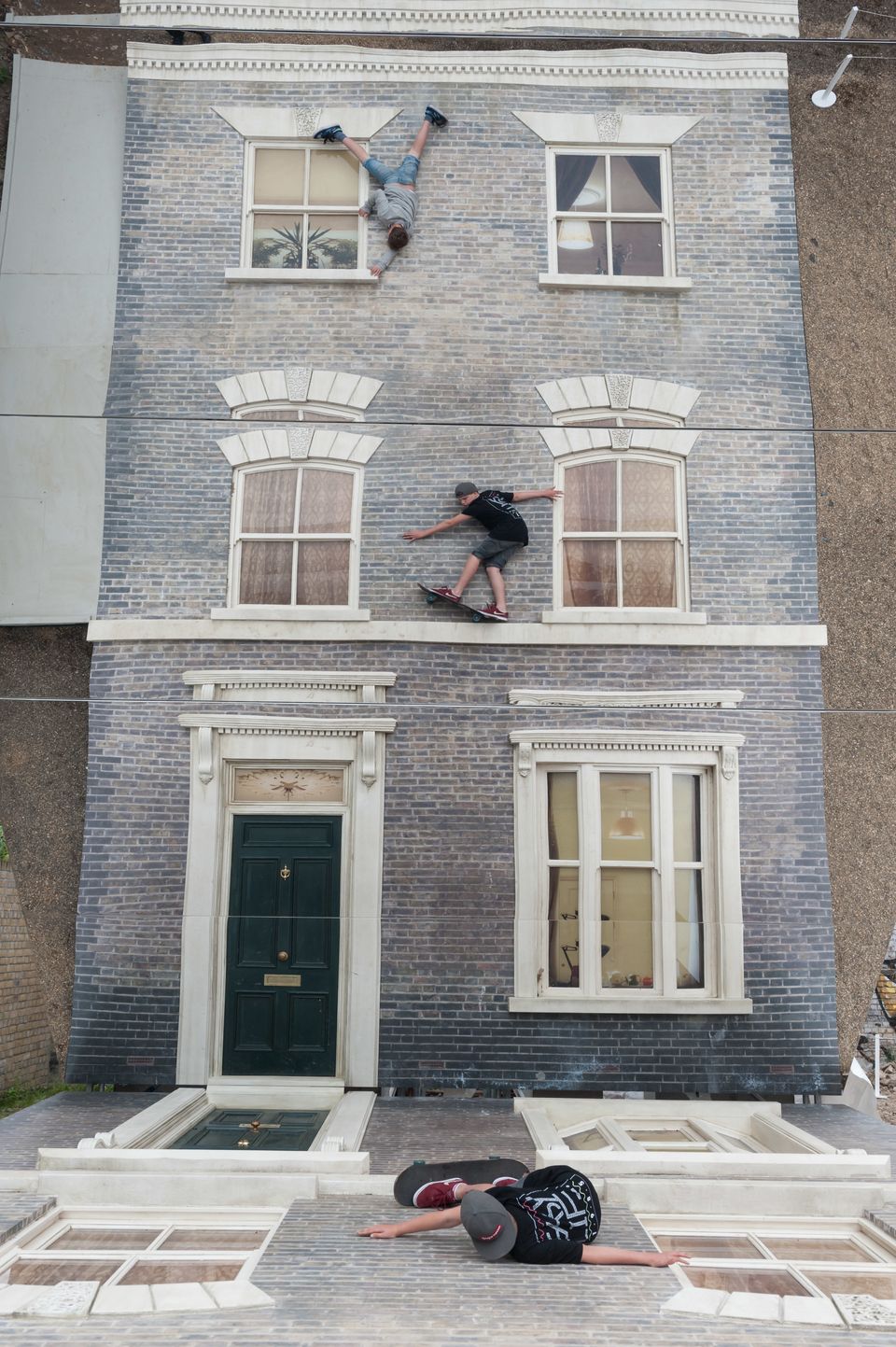In this intricate and surreal image, we see a scene that's both perplexing and artistic, giving the impression of a gravity-defying setup. The focal point is a building with a gray, white, and slightly blue brick facade, accentuated by black doors with a peephole and a brass-colored mail slot. Each window features white trim, adding to the stark contrast against the building's brickwork. 

On the wall of this building, positioned as if defying gravity, there are three people. One individual is lying on a skateboard, seemingly attached to the side of the building. He is wearing a black t-shirt and a backwards hat, giving the impression that he's looking downward, even though he's horizontal against the wall. Above, another person is upside-down, holding onto the edge of a window with their legs above the window and head down, further adding to the disorienting effect. 

To add a layer of complexity, at the bottom of the image, there appears to be a reflection or duplicated image of the building and the skateboarder, creating an abstract and mirrored perspective, making it look as if another building is directly opposite. The combination of these elements suggests a meticulous setup, possibly for a film or a creative art piece, creating an illusion that challenges the viewer's perception of reality.